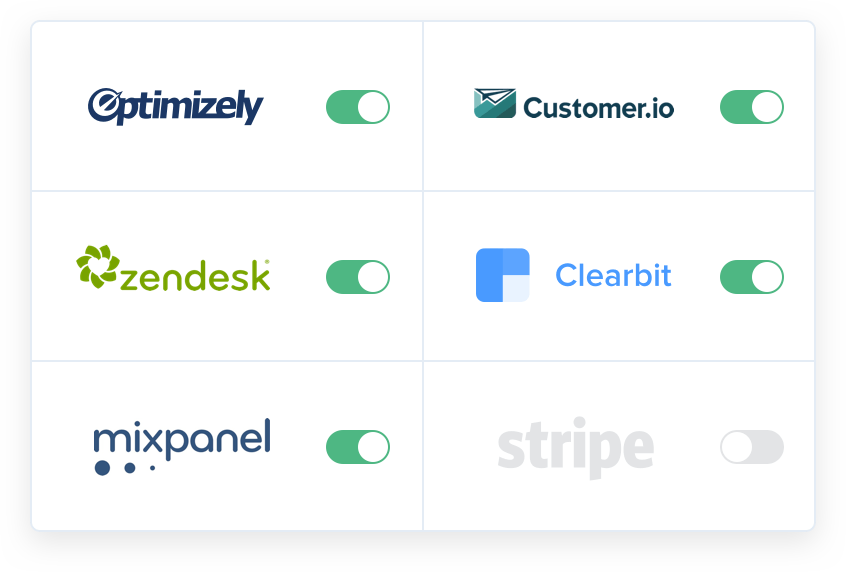The image showcases a grid of six distinct advertisements, each situated within its own light gray-bordered cell. The layout is organized into three rows and two columns, separated by vertical and horizontal lines. 

In the first row, from left to right:

1. **Optimizely**: Displayed in all blue text with a streak through it, the Optimizely advertisement features a slider button set to the right, indicating active status with a green background.

2. **Customer.io**: This ad depicts a paper airplane soaring through the air on a green background. Similar to Optimizely, the slider button is positioned to the right, marking it as active.

In the second row, from left to right:

1. **Zendesk**: Showing a green spiral-like shape with an olive hue, this ad's slider button is also slid to the right, signifying it is enabled.

2. **Clearbit**: Presenting a box with three out of four segments filled in dark blue, leaving the bottom right segment white. The Clearbit slider is set to the right, indicating it is active.

In the third row, from left to right:

1. **Mixpanel**: This ad is prominent with its navy blue color, and the slider is positioned to the right, signifying that it is active.

2. **Stripe**: Contrary to the others, the Stripe advertisement is grayed out with the text “S-T-R-I-P-E” and the slider is moved to the left, marking it as inactive.

Each ad is distinctly separated by the light gray lines that create a structured and organized visual format.